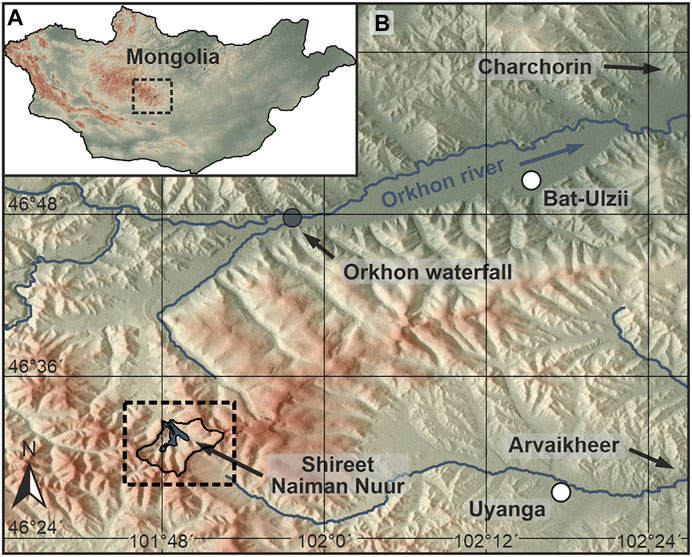The image is a detailed topographical map of Mongolia, with a two-part focus. In the top left corner, there is an inset labeled 'A,' which displays the entire country of Mongolia with a white background and a dashed line highlighting a specific area in central Mongolia. This inset provides an overview, indicating the zoomed-in section presented in the main part of the map labeled 'B.'

The main map showcases detailed topographical features of the highlighted area, emphasizing the Orkhon River and Orkhon Waterfall. It includes textured 3D renderings of contour lines colored in rust for the hills and green for lower elevations. The map also features black arrows pointing to various points of interest and landmarks, alongside longitude and latitude lines for precision. Notable labels include 'Shireet,' 'Neum,' 'Chorin,' 'Batulzii,' 'Uyanga,' and 'Arvikher,' with corresponding symbols for towns and natural features. Additionally, there is a compass rose indicating north and a section marked with another dashed box.